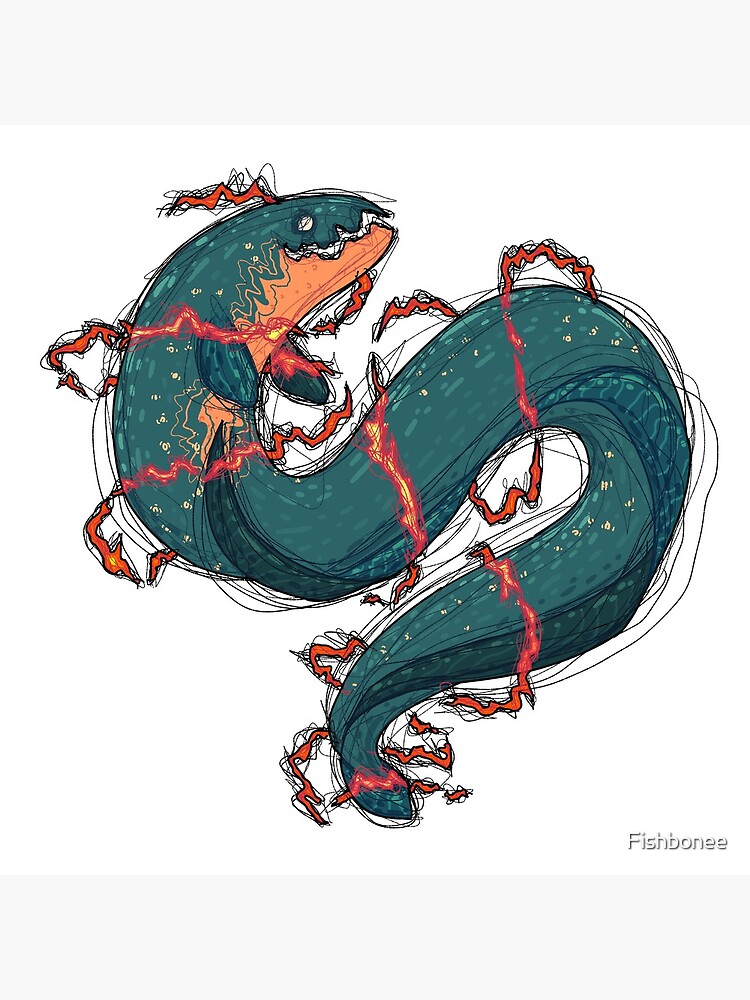The image portrays a cartoon-like sea serpent or large eel, depicted in a portrait orientation on a blank white background. The creature's head, facing right, is notable for its greenish-turquoise coloration with a light orange hue along the lower jaw and behind it. The sea serpent's body is predominantly green with yellow specks scattered throughout.

Twisting into an 'S' shape, the creature's body follows a convoluted path: starting from the head moving left, then downward, rightward, upward, rightward again, downward, and finally ending with the tail slightly down to the right. Adorning the length of the sea serpent are red ribbons and multiple black strings that intertwine over and under, suggesting dynamic movement akin to electrical zaps or fine ink lines that give the appearance of energy or fire wrapping around it.

The artwork is bordered in light gray at the top and bottom. In the bottom right-hand corner, the word "fishbone" is inscribed in white letters, with an extra 'E' at the end, perhaps signifying the name of this fantastical, undulating creature. The design evokes the imaginative creation of a youthful artist, brimming with vibrant colors and intricate details.